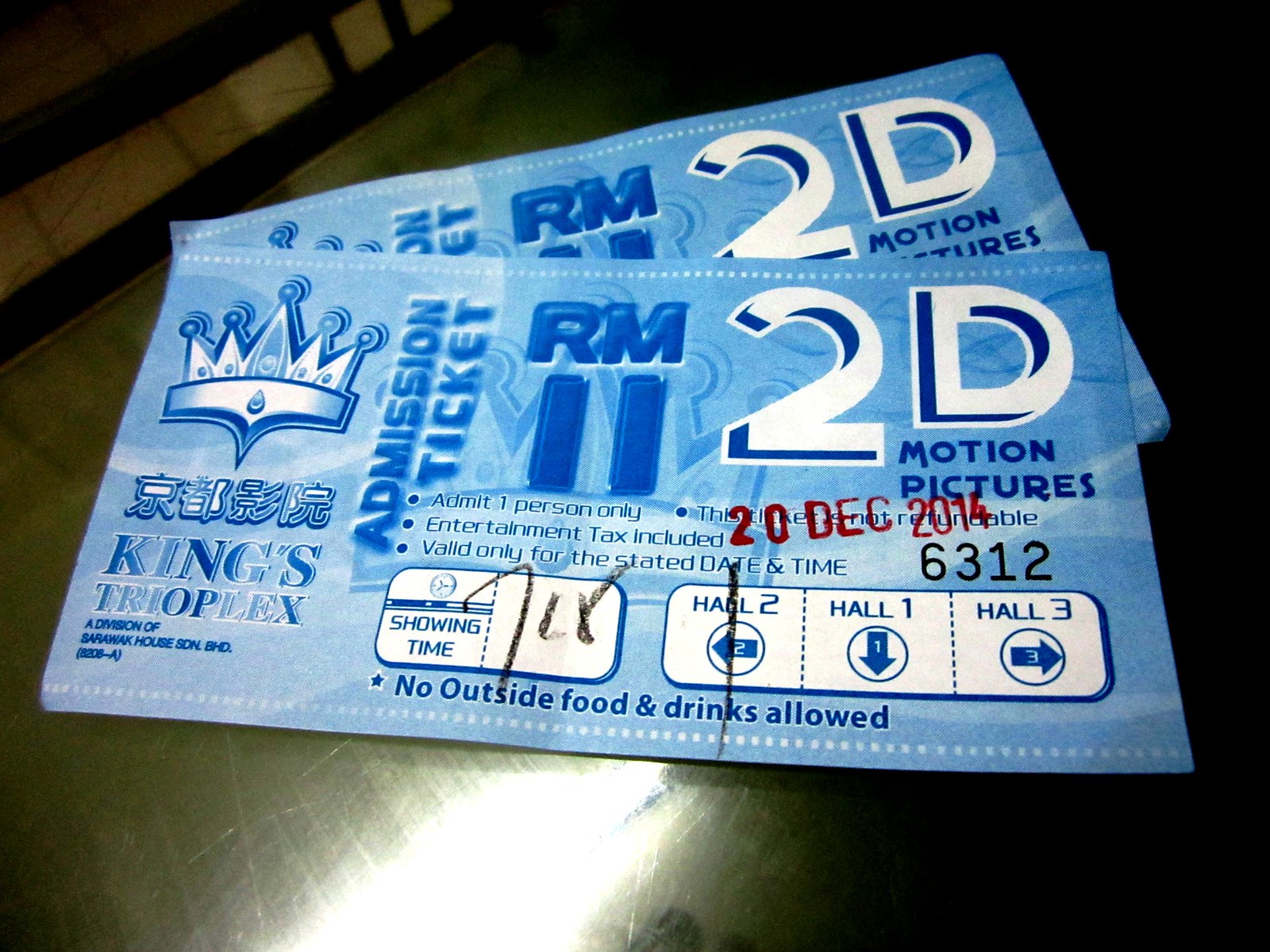The image shows two almost identical admission tickets lying on top of each other on a hard, shiny surface that reflects light. The tickets are light blue with darker blue and white text. Dominating the top of each ticket is an off-color blue crown with some Japanese or Asian lettering underneath. The primary text reads "King's Trioplex," and below that, "admission ticket" is printed vertically. Each ticket indicates "RM-11 2D motion pictures," and specifies "Admit one person only," "Entertainment tax included," and that it is "Valid only for the stated date and time." The date "20 December 2014" is stamped in red ink, with the serial number "6312" in dark black. Besides, there is a box marked "showing time 7/18." The tickets also have arrows pointing to "Hall 2," "Hall 1," and "Hall 3," emphasizing no outside food and drinks are allowed.